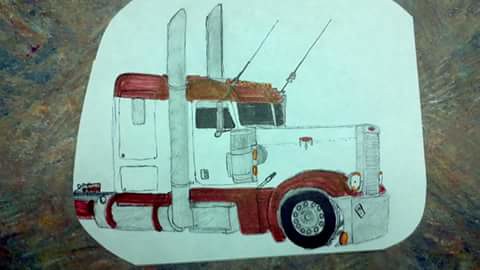The image showcases a meticulously crafted drawing presented in a rectangular, landscape format. This drawing is situated on an irregularly shaped oval piece of pristine white paper, which lies atop a textured, marble-like stone surface exhibiting a blend of brown, blue, and gray hues. The focal point of the drawing is the striking front view of a semi-truck, adorned predominantly in white with bold red accents along its edges. The truck is detailed with substantial front wheels and two distinct antennas extending from its top. Additional features include two metal rods positioned on either side just behind the doors, each protruding upwards beyond the truck's roof, adding a touch of industrial realism to the artwork.